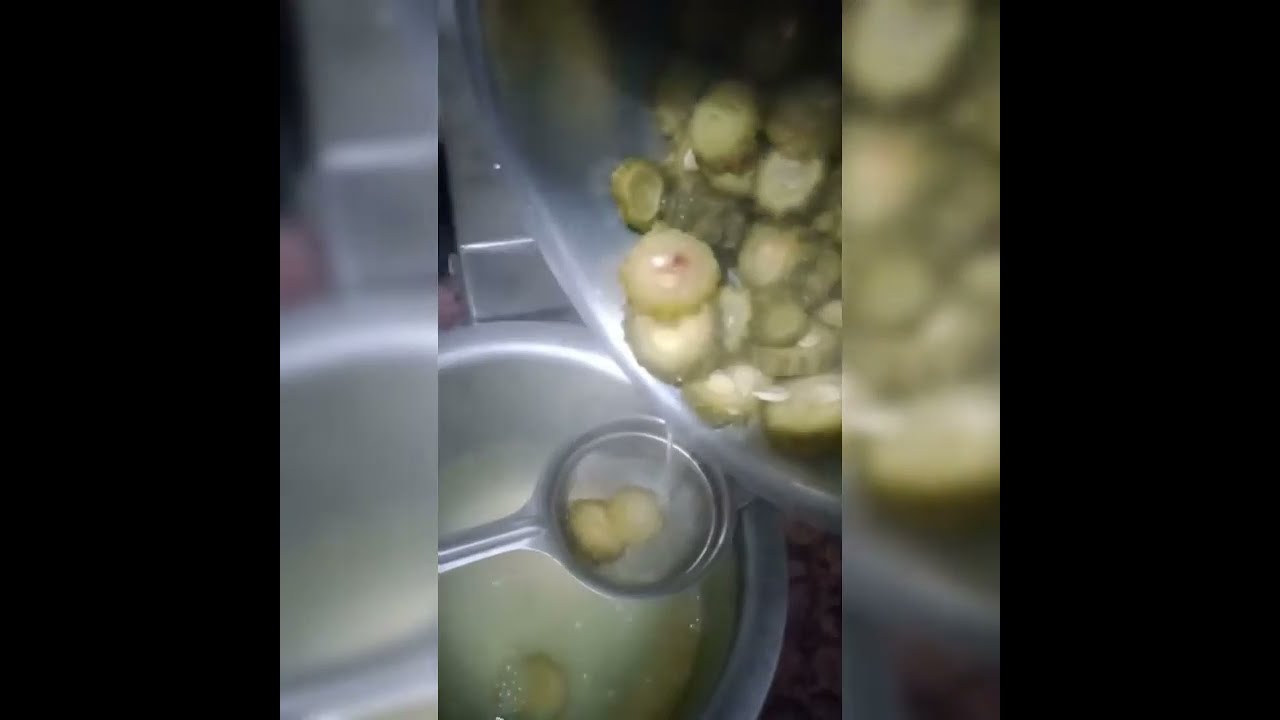The image is a close-up, vertical shot taken by a cell phone, featuring a metal pot, which is dull chrome in color, resting on the corner of a stove that appears to be gas-operated. The image centrally showcases the pot's contents from an overhead angle, revealing a mixture of vegetables, possibly onions or potatoes, and other green vegetables submerged in water. The pot is filled with about 20 circular-shaped vegetables, with most remaining whole and some sliced, emitting a steam that veils the white marble tile backsplash in the background. The main image is framed by faded and blurred repetitions of itself on either side, creating a square shape. This central square is flanked by two black rectangles, extending the overall aspect ratio to a wide format. The entire composition conveys a sense of culinary preparation in a sleek kitchen setting.